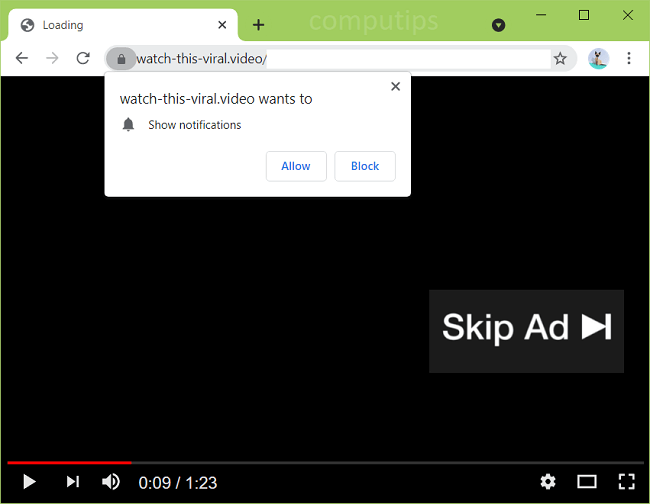The image captures a computer screen in the middle of loading a webpage. A prominent pop-up box takes center stage, commanding attention with the prompt "Watch this viral video." Below this prompt, the text is reiterated with the same phrase, "Watch this viral video," creating a redundant emphasis. The pop-up box also includes options to either "Show notifications" with clickable buttons to "Allow" or "Block" these notifications. In the upper right corner of the pop-up, a small 'X' is present for closing the box.

In the lower right-hand corner of the screen, a "Skip Ad" button is visible, accompanied by a small arrow pointing downward, suggesting an interactive feature for viewers to bypass the advertisement. Just above this, the video player interface is partially visible, revealing that the video is nine seconds into its duration of 1 minute and 23 seconds. The progress is indicated by a red timeline bar just above the playback controls.

The controls include a play/pause button, a volume control icon, and settings options. Additionally, buttons for toggling between full-screen and half-screen modes are situated at the far-right side of the control panel. The overall scene depicts a typical user experience on a video-sharing platform, highlighting various interactive elements designed to engage the viewer.